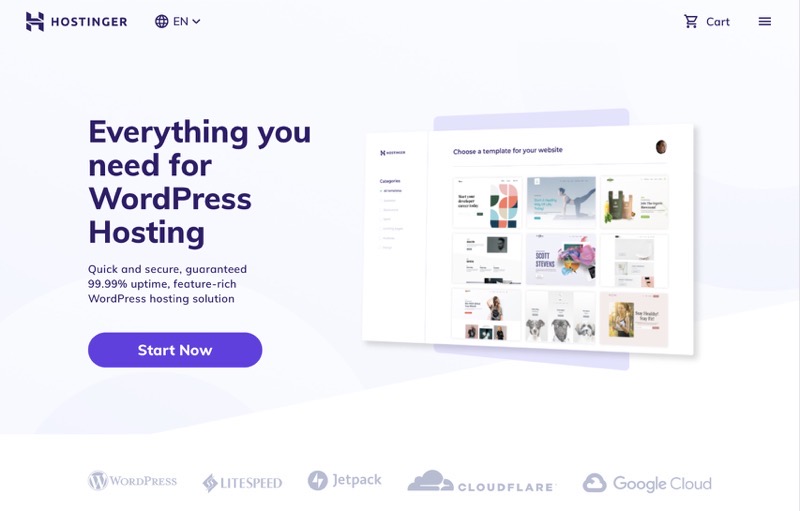This horizontally-aligned image showcases a company's webpage, viewable on both computers and smartphones. The background presents a subtle ombre effect in shades of light white, blue, and purple, blending seamlessly to create a soft, pale backdrop.

In the upper left corner, there is a small "H" symbol followed by the text "Hostinger". Adjacent to this is a world icon indicating that English is the selected language. Moving to the upper right corner, you’ll see a shopping cart icon with the word "Cart" next to it, along with a horizontal line which serves as a more options menu button.

Dominating the left-hand side is a bold headline that reads, "Everything you need for WordPress hosting". Directly below this, in a slightly smaller font, is the text, "Quick and secure, guaranteed 99.99% uptime, feature-rich WordPress hosting solution." Beneath these lines is a prominent purple "Start Now" button, encouraging users to begin their journey.

To the right of the textual descriptions, there is an illustration of a computer screen to visually represent the services described. Below these main elements, several icons aligned horizontally denote additional features and integrations: WordPress, Lightspeed, Jetpack, Cloudflare, and Google Cloud.